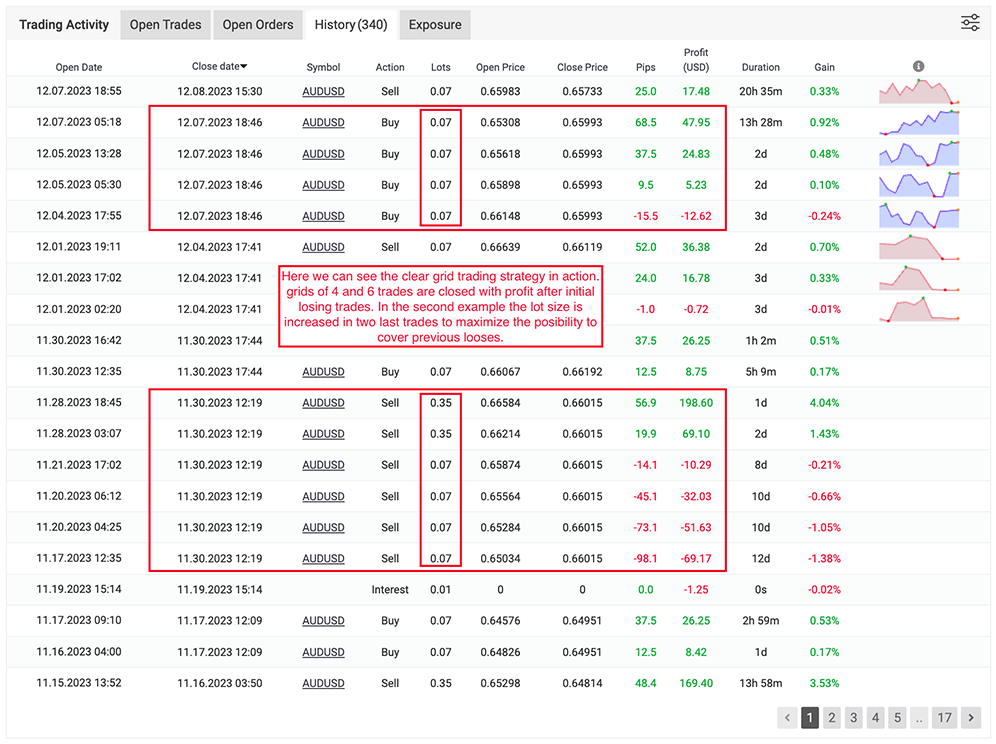The image is a large and detailed screenshot of a spreadsheet-like interface. At the top of the screen, there are several tabs labeled: "Trading Activity," "Open Trades," "Open Orders," "History (340)," and "Exposure." In the middle of the screen, there's a text box containing the following message: "Here we can see the clear grid trading strategy in action. Grids of 4 and 6 trades are closed with profit after initial losing trades. In the second example, the lot size is increased in the last two trades to maximize the possibility of covering previous losses." This interface seems to be a comprehensive tool for managing and analyzing trading activities, highlighting strategic decisions within a grid trading approach.